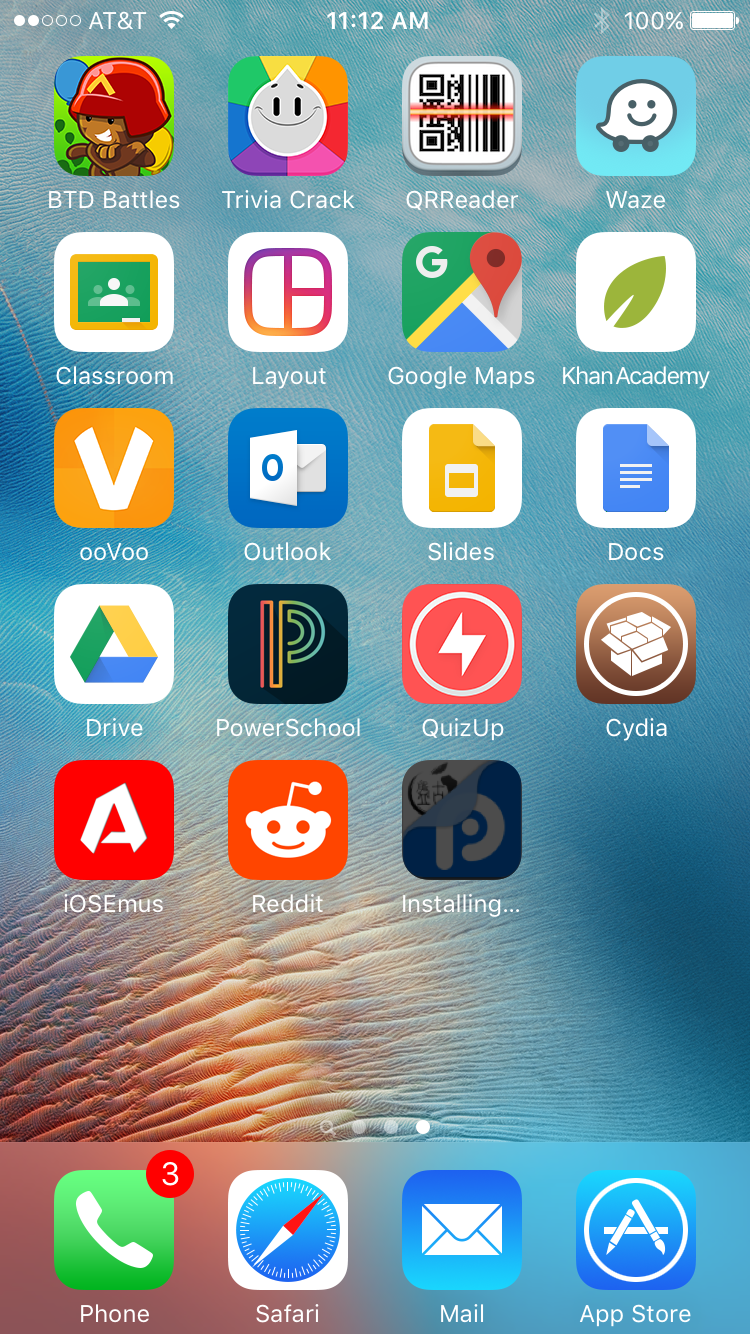The image depicts the home screen interface of an Apple iPhone. In the top left corner, the carrier information shows "AT&T," while the center of the status bar displays the time as "11:12 a.m." In the top right corner, the battery is fully charged at 100%, with a small Bluetooth icon next to it.

Beneath the status bar, the screen is filled with app icons arranged in a grid. Starting from the top left, the visible app icons are as follows: BTD Battles, Trivia Crack, QR Reader, Waze, Classroom, Layout, Google Maps, Khan Academy, OOVOO, Outlook, Slides, Docs, Drive, Power School, QuizUp, Cydia, iOS Emos, Reddit, and a final icon indicating an app currently installing.

At the bottom of the screen, there are four docked icons: the Phone app with a red notification badge displaying the number three, Safari, Mail, and the App Store.

The phone's background features an abstract design with blue and orange hues, resembling sand. Each app icon vividly represents its function through distinctive graphics.